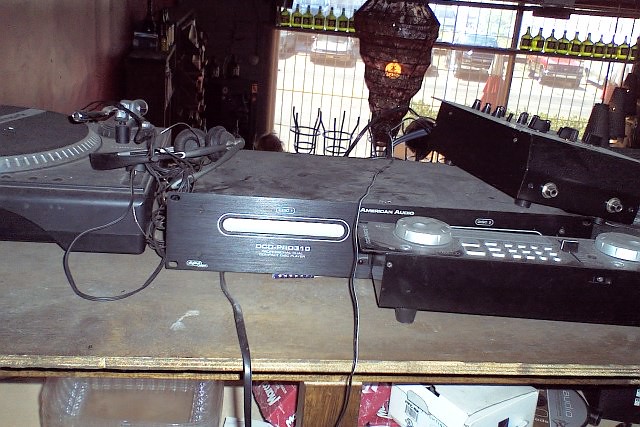In this image, we are inside what appears to be a bar or a business setting that is not currently open for the day. Prominently featured in the foreground is a rough plywood table displaying various pieces of audio equipment. On the far left side of the table, there is a dark gray turntable with the needle placed off to the side. Next to it, there is a pair of headphones and what looks like a hi-fi audio unit, identifiable by its volume gauges and several silver circular components. Further to the right, there is more audio equipment, including a mixing console with multiple knobs and sliders, possibly used by a DJ, along with visible cords and wires. Beneath the plywood table, there is cluttered storage, including plastic containers and other miscellaneous items.

In the background, the setting resembles a bar with barred windows illuminated by bright sunlight, allowing a view of vehicles parked outside. On the shelves against the windows, there are bottles filled with a yellow liquid, likely alcohol. Additionally, some silver-toned metal bar stools are stacked upside-down, contributing to the atmosphere of a bar prepping for business hours. The overall scene combines elements of both a bar and a DJ setup, filled with various dusty, older electronic audio equipment designed for mixing and playing music.